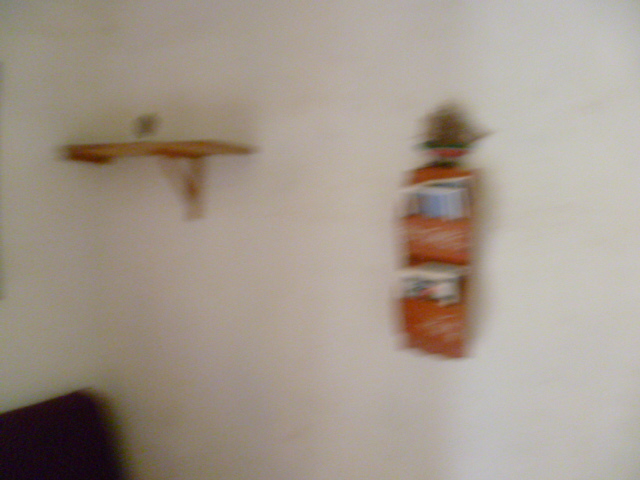This is a very blurry color photograph taken inside a dimly lit room, likely someone's living room. The white or light gray walls are difficult to discern due to the lack of focus. On the far left side of the image, there's a small wooden shelf supported by a bracket. Adjacent to it, several feet to the right, there is a brown or red magazine rack that holds mostly white-colored magazines; there's also an indiscernible saying on it. At the top of the rack, there's a decorative element—perhaps a small planter or an emblem. The bottom left corner of the image reveals part of a dark-colored cushion, possibly dark blue or dark black, which might belong to an armchair or couch. Additionally, an orange rectangular decoration with green and red ribbon can be seen hanging on the wall. Despite the poor quality and dim lighting, details like the wooden shelves, magazine rack, and wall decorations can be faintly made out.